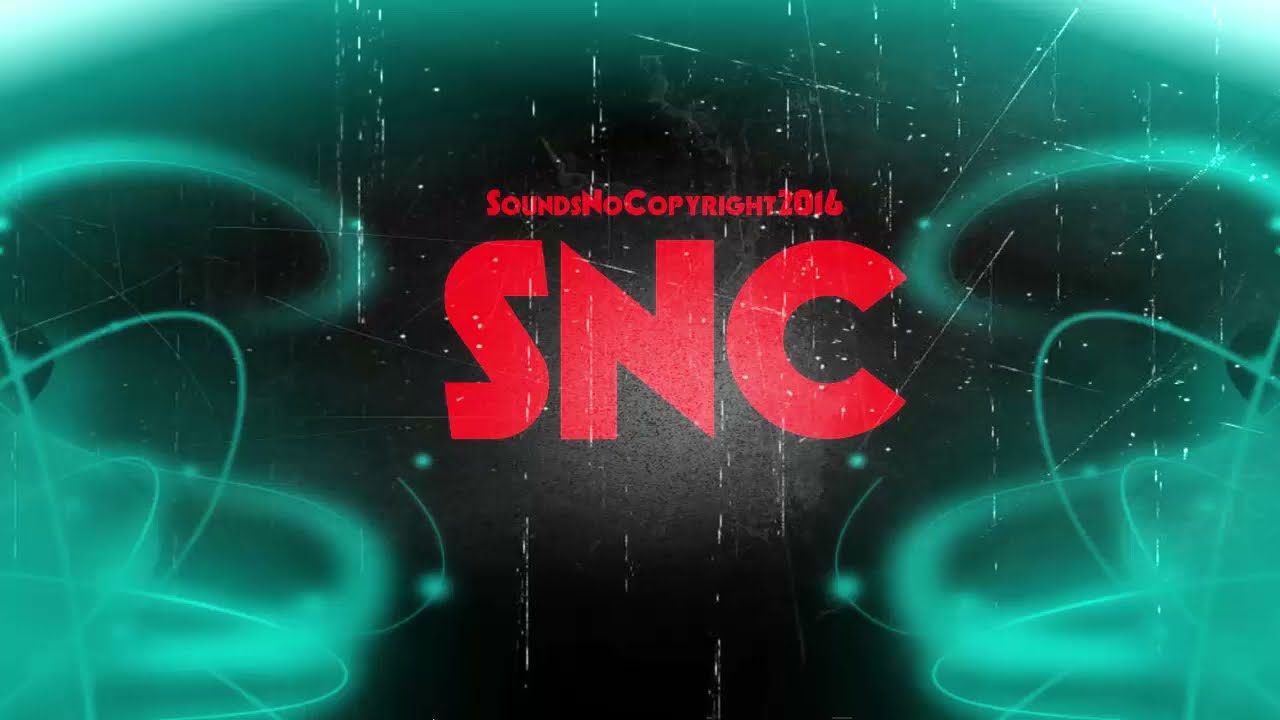The image appears to be designed for either a video or an advertisement. It features a vibrant black background accented with bright, electric blue glows around the edges. In the center, a bold red font reads "Sounds No Copyright 2016," with the letters "SNC" displayed prominently just below in an even larger red font. The backdrop includes swirling and glowing patterns of green and blue, with additional white scratch-like lines scattered throughout, adding to the dynamic and electric aesthetic. The overall effect is a highly colorful and eye-catching composition, suitable for music or media-related content.